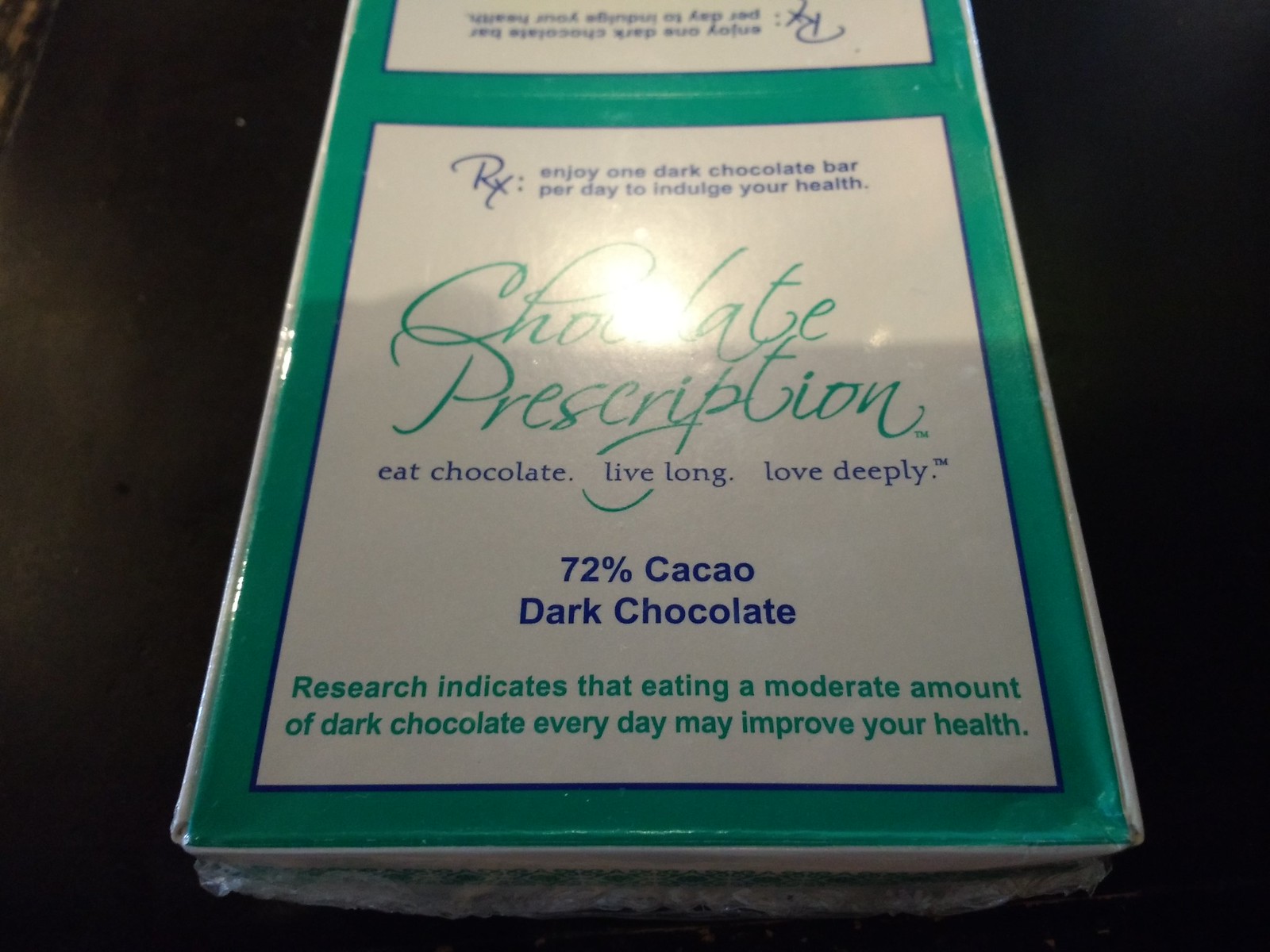This photograph features a green-colored box designed for chocolate, placed on a flat white tabletop background. The box has a matte finish and minimal details, except for a prominent square white label bordered in blue. Inside the white box, blue print reads: "Rx, enjoy one dark chocolate bar per day to indulge your health." The label also includes green text that reads "Chocolate Prescription," and further blue text stating "Eat chocolate, live long, love deeply, 72% cacao dark chocolate." Additionally, green lettering at the bottom of the label provides a note: "Research indicates that eating a moderate amount of chocolate every day may improve your health."